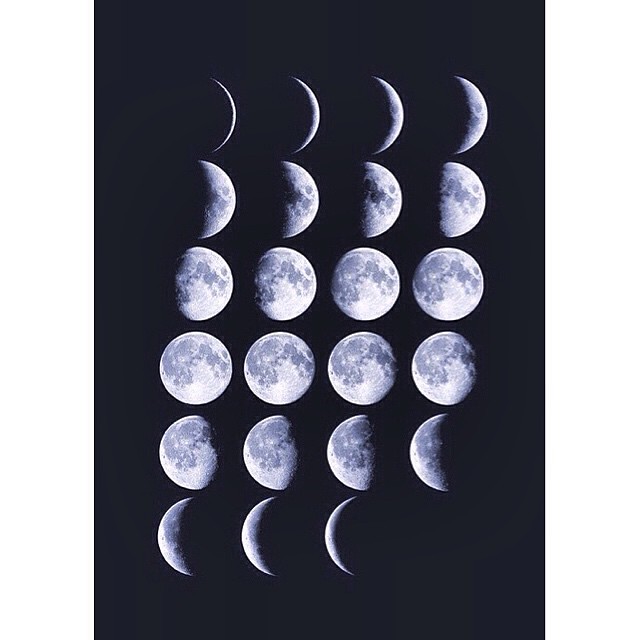This image exhibits the phases of the Moon, depicted in a striking black-and-white format. The photograph has a black background and showcases six rows of Moon images, with four images per row. Starting from the top row, the sequence begins with a new Moon in varying stages, gradually becoming more illuminated. By the time it reaches the second row, the crescent Moon evolves into a half Moon, continuing to wax into a waxing gibbous Moon. The third row sees the Moon approaching near fullness, culminating in a full Moon displayed predominantly in the fourth row. As the sequence progresses downward, it captures the Moon transitioning from a full moon to a waning gibbous in the fourth and fifth rows. The last two rows depict the Moon increasingly shadowed, transitioning towards the final stages. The fifth row covers the descent to a half moon, while the sixth row showcases the Moon diminishing into a waning crescent, ultimately fading to a small sliver, and finally disappearing completely. The photograph's only hues are various shades of black, white, and gray, highlighting the lunar phases without any accompanying text or additional elements.